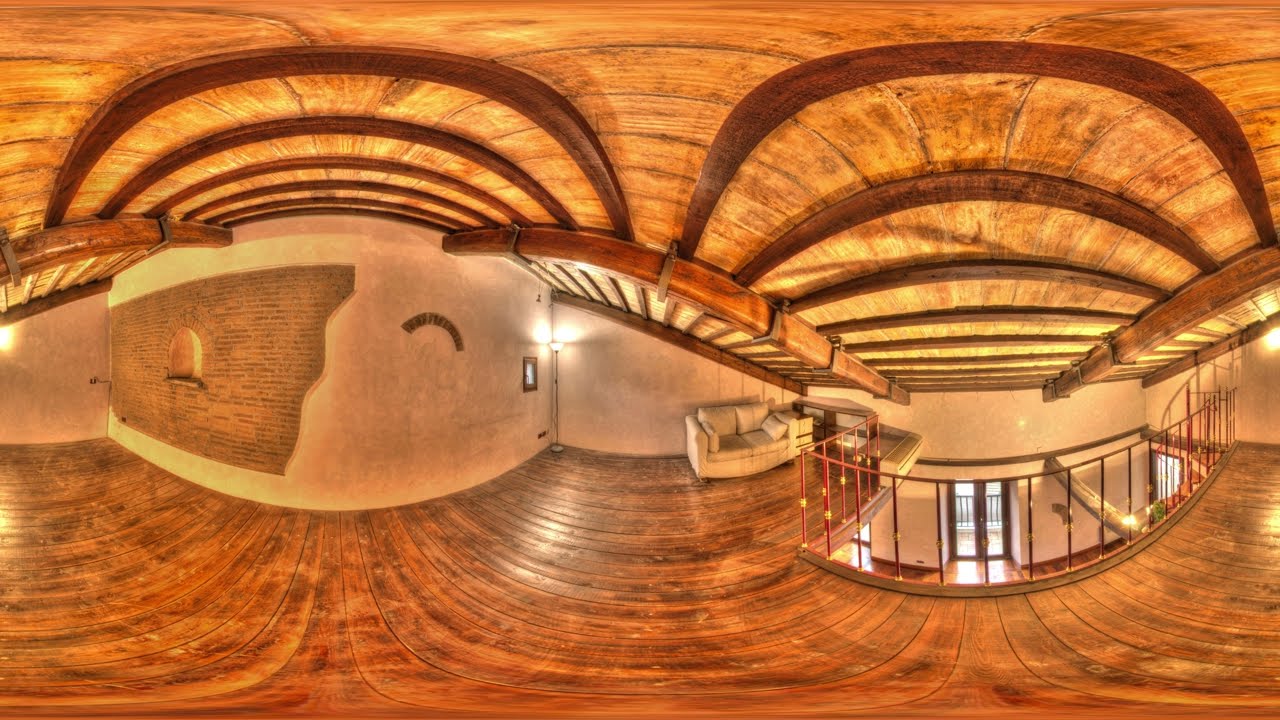This image, captured with a fisheye lens, depicts the cozy, rustic interior of a large wooden building with a warm, inviting ambiance. The second floor features wooden floors and ceilings, as well as exposed wooden beams and supports that enhance the space's aged, earthy feel. The walls are primarily stucco or plaster, with sections revealing a small brick cutout that resembles an old kiln or brick oven. A leather love seat is thoughtfully placed next to a lamp and a little shelf, adding to the relaxed vibe of the space. 

From the upstairs perspective, a small window and a red railing with gold accents can be seen, leading to a staircase descending to the lower floor. This lower floor, visible from the balcony, continues the rustic theme with the same ancient wooden aesthetic. Christmas lights twinkle downstairs, contributing a festive touch, and through one of the downstairs doors, the image reveals a sunny day outside. The entire scene is bathed in warm brown tones from the extensive use of wood, creating a laid-back and peaceful atmosphere perfect for unwinding and enjoying the serene environment.